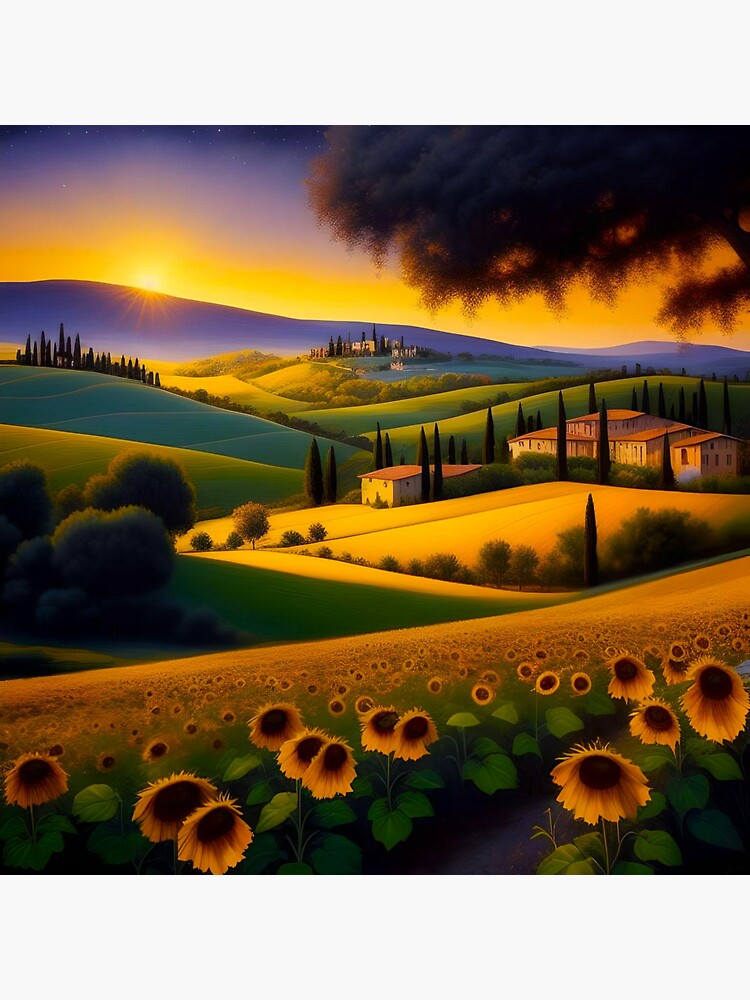This square, computer-generated image depicts a vibrant and detailed rural scene during a sunset, merging artistic styles to create a cartoonish yet picturesque atmosphere. The foreground is dominated by a field of sunflowers in full bloom, their orangish-yellow petals and black centers set against robust green stalks. The sunflowers stretch across the entire bottom half of the image, transitioning from large, individually distinct flowers near the viewer to a seamless golden sea as they recede into the distance.

Beyond the sunflower field lies a patchwork of farm fields, including a golden wheat field and verdant green sections, interspersed with tall trees and scattered shrubs. Nestled among these fields are several houses that feature distinctive white walls and red gabled roofs. Particularly notable is a larger Tudor-style house surrounded by smaller buildings, which adds to the idyllic rural ambiance.

In the background, rolling green hills and purple-tinged mountains create a layered horizon, with the sun setting behind them, casting a warm, orangish hue over the clear sky. To the left, a cluster of city towers can be faintly seen, while the top middle and right parts of the image include blurred tree outlines, adding depth and framing the sunset scene.

Overall, this detailed, pastoral landscape combines natural beauty with rural architecture, capturing the serene transition from day to night in a pastoral setting.